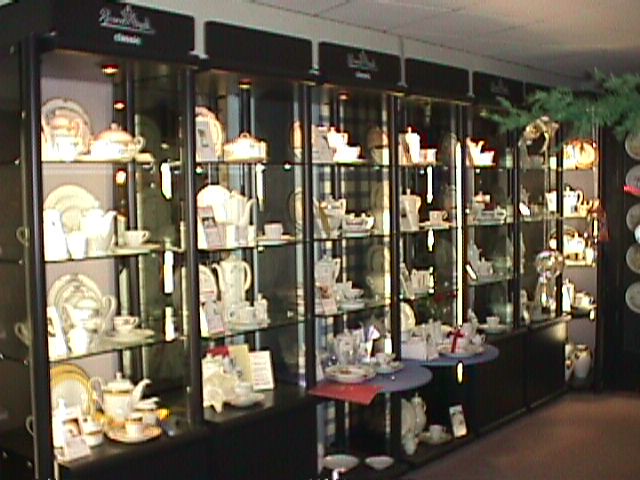The image depicts the interior of what appears to be either a luxurious home display or an exclusive antique shop. The scene features a variety of ornate and sophisticated items such as tea kettles, plates, cups, silverware, and chinaware, all meticulously arranged in glass boxes or on shelves. The overall design is elegant and clean, with a dominant white color palette accented by hints of gold in the lower left corner. These items seem to be purely decorative, suggesting they are not intended for regular use but rather to showcase their intricate design and high value. The arrangement of the pieces is both neat and aesthetically pleasing, exuding an air of refined taste and exclusivity.